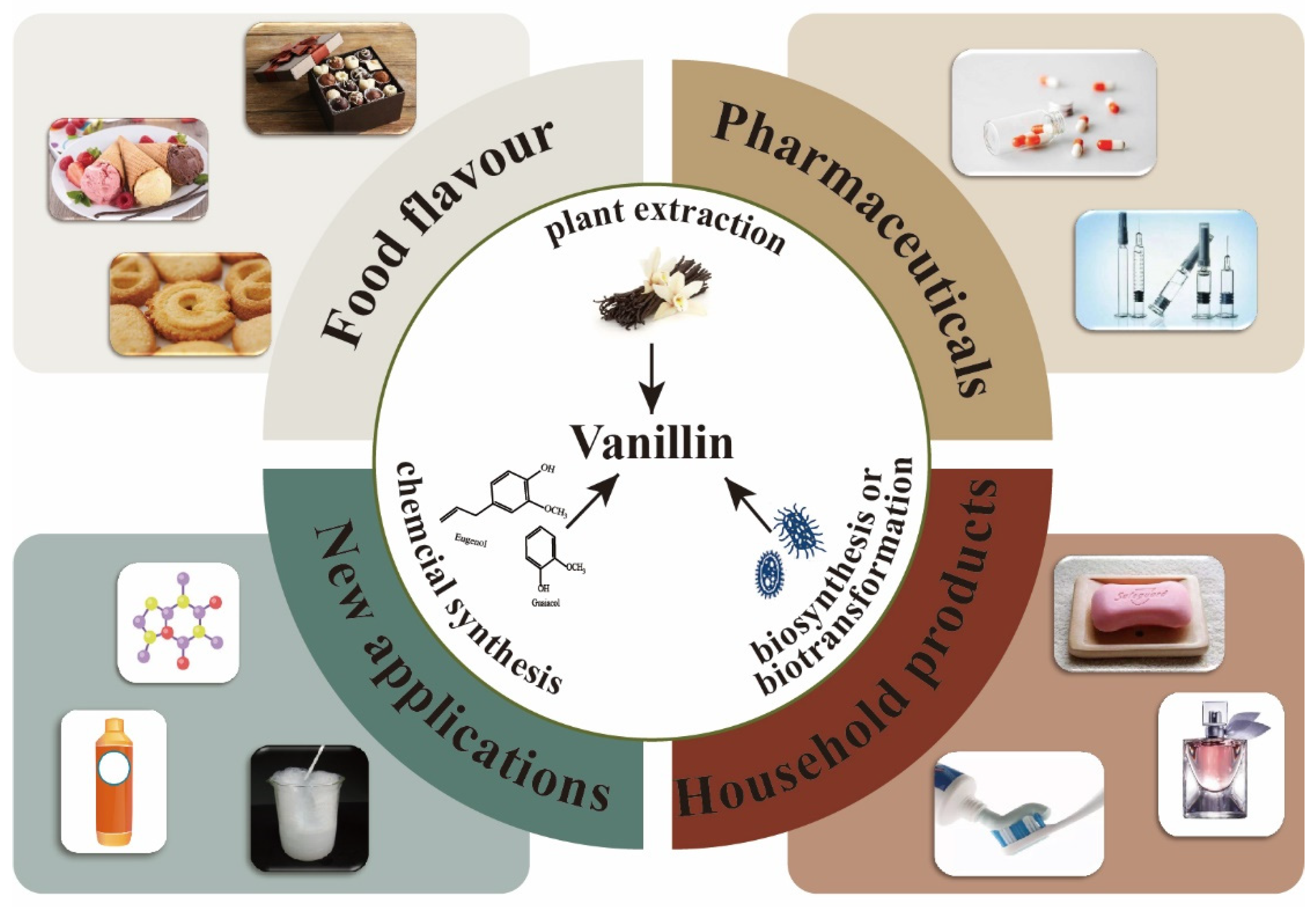The image is a detailed, digitally-created diagram, resembling a PowerPoint slide, that illustrates the various uses and production methods of vanillin, a compound derived from vanilla. Central to the image is a large white circle segmented into four parts, each describing a different method of vanillin production: "Plant Extraction" at the top, "Chemical Synthesis" to the left featuring chemical cells, and "Biosynthesis or Biotransformation" to the right depicting blue cells. An arrow from a picture of vanilla beans points downward to the term "vanillin" in the center.

Surrounding this central circle are four outer sections, each depicting a major application of vanillin. In the top-left section labeled "Food Flavor" (gray), images illustrate the use of vanillin in chocolates, cookies, and ice cream cones with chocolate, vanilla, and strawberry flavors. Moving clockwise, the top-right brown section labeled "Pharmaceuticals" shows pills, vials, and syringes, highlighting vanillin's role in this field. The bottom-right maroon section, "Household Products," includes icons of soap, toothpaste, and perfume, showcasing vanillin's application in everyday products. Finally, the bottom-left green section, labeled "New Applications," depicts a diagram of chemical molecules, a canister, and a cup with white foam and a spoon, suggesting innovative uses for vanillin.

Each application is visually represented by detailed images: food items in the top box, scientific equipment and designs in the left box, medical supplies in the right box, and household products in the bottom box. This comprehensive layout underscores the versatility and widespread utility of vanillin across various industries.